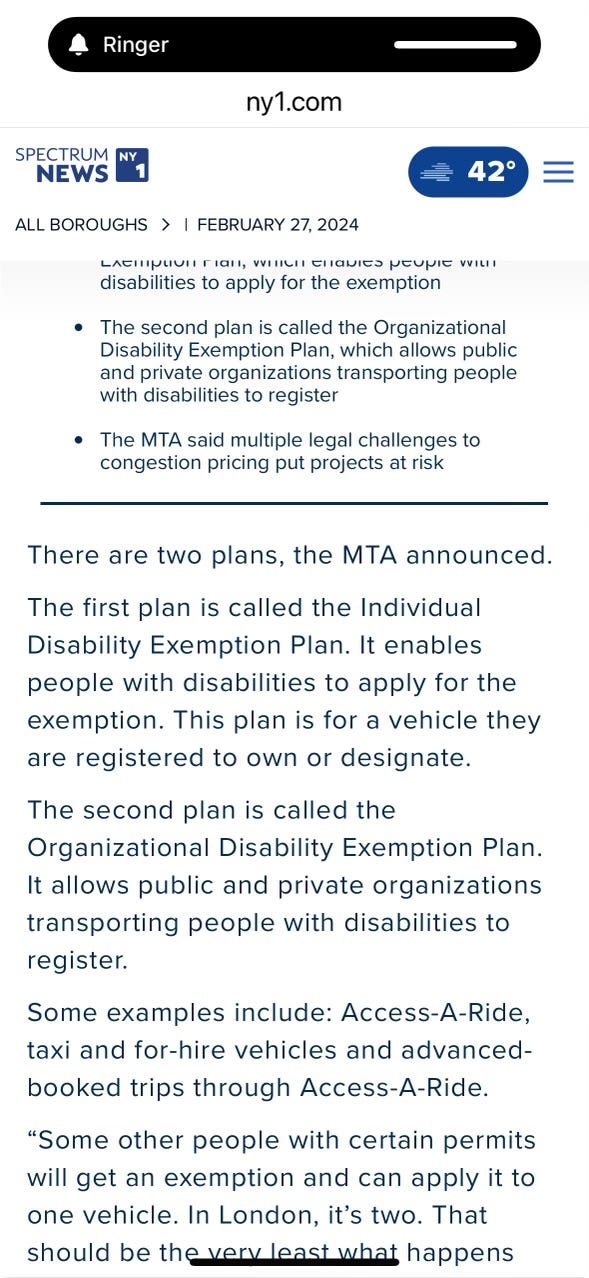The image depicts a mobile-optimized web page from ny1.com, featuring Spectrum News. At the top center, a black search box with a white bell icon and the word "Ringer" is visible. The logo of Spectrum News NY1 is on the left side, with the temperature reading "42 degrees" next to it. To the right, there is a blue button and a hamburger menu labeled "All Boroughs," alongside the date "February 27th, 2024."

Beneath this, the web page mainly contains black text on a white background. The content begins with bullet points, though the top line is partially cut off, mentioning "disabilities to apply for an exemption." The subsequent point mentions the "Organisational Disability Exemption Plan," which allows public and private organizations to transport people with disabilities.

Additionally, the MTA has stated that multiple legal challenges to congestion pricing could jeopardize their projects. A black horizontal line separates this section from more detailed descriptions of the two plans the MTA announced:

1. **Individual Disability Exemption Plan**: Allows individuals with disabilities to apply for an exemption for a vehicle they own or designate.
   
2. **Organisational Disability Exemption Plan**: Permits public and private organizations, including Access-A-Ride, taxis, for-hire vehicles, and pre-booked trips through Access-A-Ride, to register for transporting people with disabilities.

The text further suggests that certain individuals with specific permits may receive exemptions for one vehicle, in contrast to London's allowance for two. Unfortunately, the closing quotation mark of this statement is cut off. Additionally, a small black band spans a third of the way across the bottom center of the screen, obscuring some of the text.